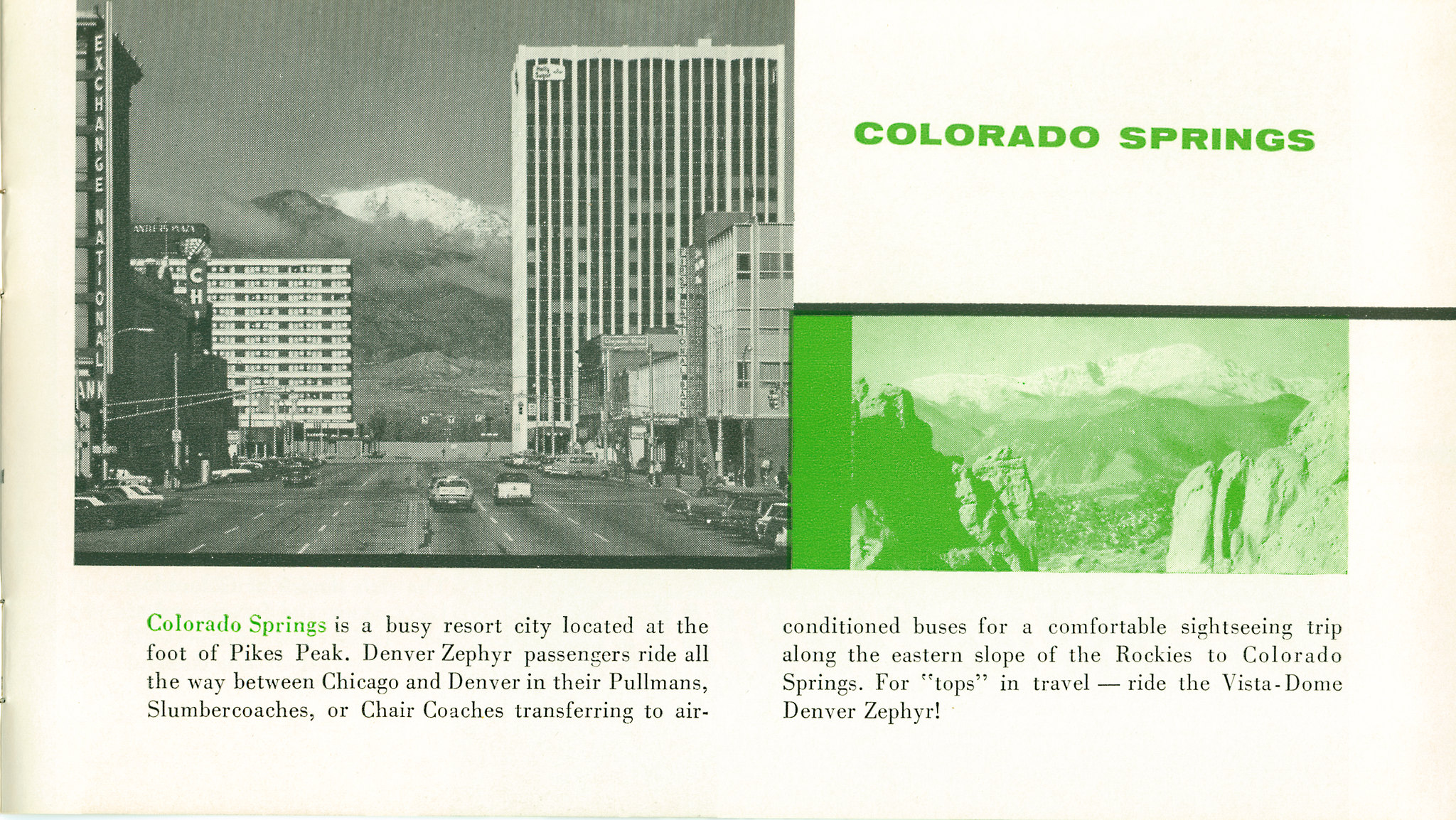This image is a page from a magazine showcasing Colorado Springs. In the upper right corner, the title "Colorado Springs" is prominently displayed in green font. Below this title are two photographs. The first photo, on the left, is a black-and-white image capturing a bustling cityscape with a prominent street running down the middle and mountains majestically rising in the background. The second image, on the right, is tinted in a bright green hue and features towering cliffs with distant mountains creating a dramatic landscape.

Underneath these images, the caption continues in green font with "Colorado Springs," followed by detailed black text explaining the location as a busy resort city situated at the foot of Pikes Peak. It describes the city's connection for passengers traveling between Chicago and Denver, highlighting the options of slumber coaches or chair coaches that transfer to air-conditioned buses for a comfortable sightseeing journey along the eastern slope of the Rockies to Colorado Springs. The text also promotes the Vista Dome, Denver Zephyr for an exceptional travel experience.